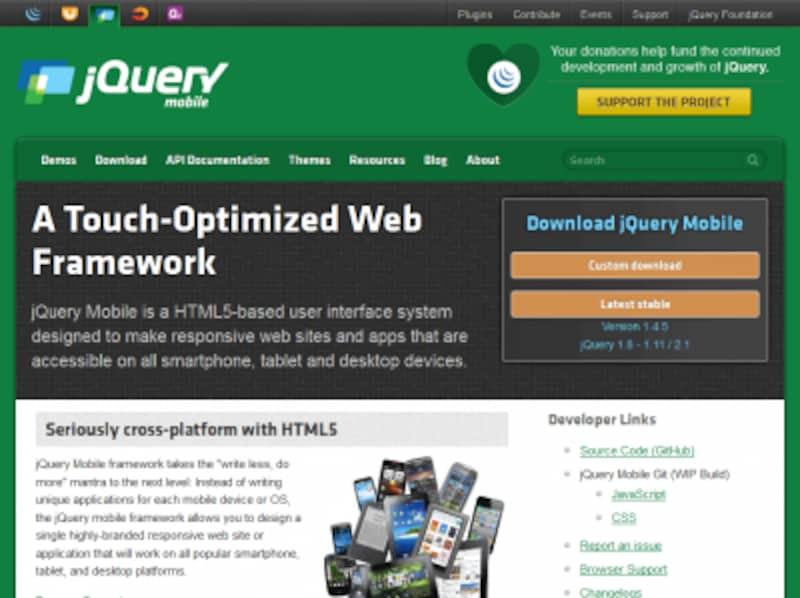A screen capture of a website is displayed, featuring a dark grey horizontal navigation bar at the top. On the upper left corner of the page, several colorful icons in blue, yellow, green, orange, and purple are visible. Directly below these icons, the text "jQuery Mobile" appears in white. On the upper right side, there is a prominent yellow rectangular button with the text "Support the Project" written on it. The backdrop of the web page is a rich, deep green.

Within the main webpage, a secondary window is set against a black and white background. On this window, located on the right side, there are two orange rectangular buttons. Above these buttons, the text "Download jQuery Mobile" is written in blue. This detailed layout hints at a sophisticated and user-friendly interface designed to promote and support the jQuery Mobile project.